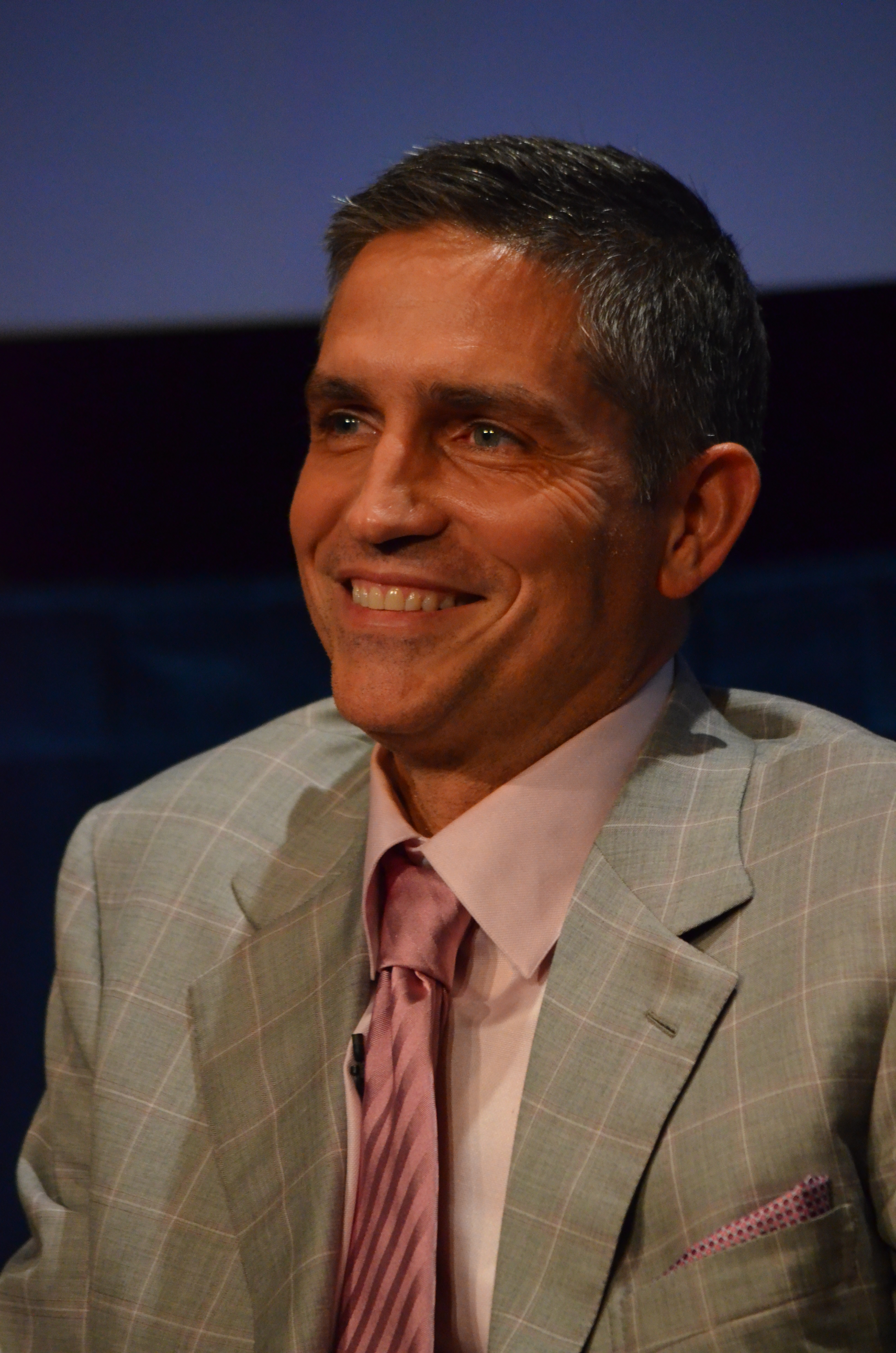The photograph features a smiling man in his mid-40s to 50s with tanned skin and short, cropped dark hair, slightly longer on top than on the sides. He has a broad grin that reveals his pristine white teeth, and the crinkles at the corners of his eyes accentuate his smile. The man, who bears a resemblance to actor Jim Carrey, is turned slightly towards the viewer's left, his gaze directed off to that side.

He is dressed in a sharp, gray checkered suit jacket with fine pink lines forming a grid pattern, complete with lapels and a visible buttonhole on the right lapel. His ensemble includes a light pink dress shirt paired with a darker pink tie featuring diagonal stripes, exuding a sophisticated yet vibrant style. A neatly folded pink pocket square peeks out from his right breast pocket, adding a touch of elegance.

The background, though out of focus, is a gradient of colors starting with a dark section at the bottom, transitioning to medium blue, and finally to a deep purple at the top. This gradient is aligned slightly diagonally with the higher side on the right. The overall look of the photograph suggests a timeless style, influenced by fashion trends from the late 1980s to early 2000s.